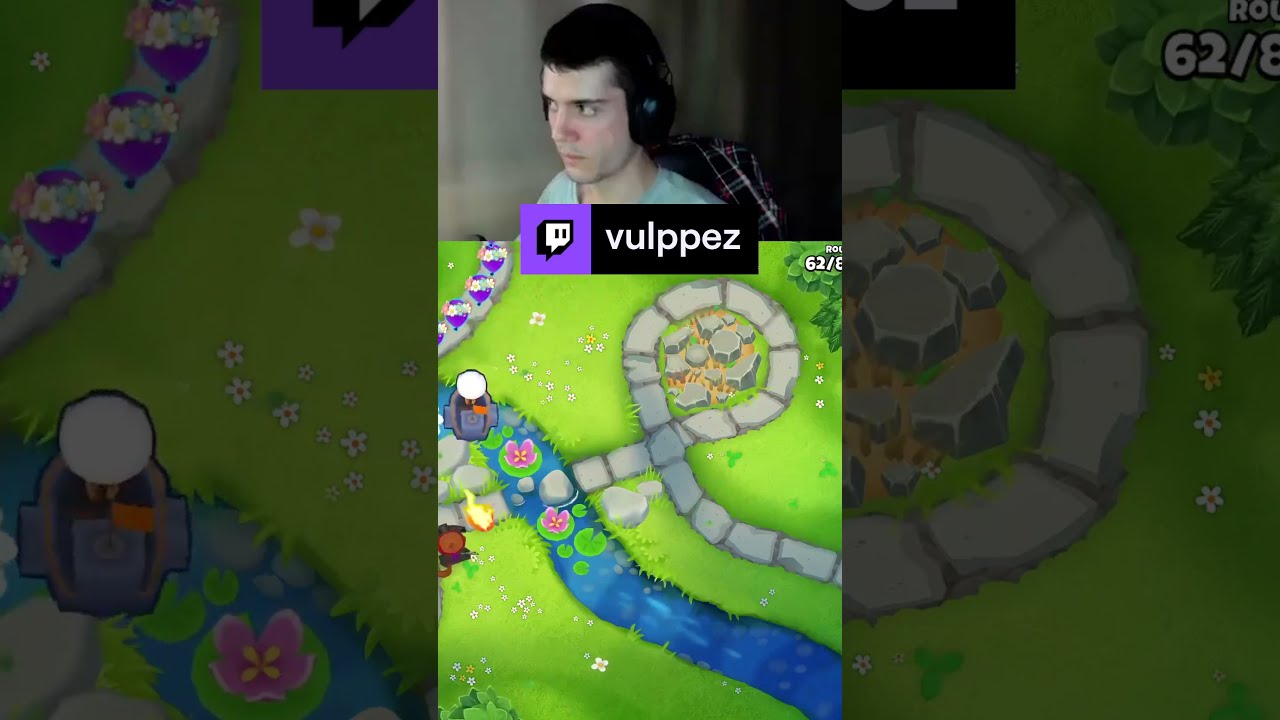The rectangular image, approximately six inches wide and three to four inches tall, appears to be a screenshot from a video game. The image is divided into three sections: left, center, and right. Dominating the center upper portion is a small photograph of a man, presumed to be in his mid-twenties with short dark brown hair, wearing over-the-ear headphones and a flannel shirt draped over the back of his chair. The man seems slightly aggravated, possibly due to the game he is playing, evident from his side-eye glance.

Below his picture, there's a distinctive logo reading "VULPPEZ" accompanied by a little ghost figure to its left and a purple square with a white speech bubble containing eyeballs. This suggests the image is from a streaming platform, likely Twitch, indicated also by the viewer count section appearing faintly in the top-right corner.

The actual game depicted in the image shows an aerial view of a vibrant green meadow bisected by a blue river flowing from the bottom right to the top left. The river features stepping stones, lily pads, and flowers. On the left side of the stream, there’s a small campfire setup. Central to the meadow is a circular stone path that forms a rock maze, looping around a central stone monument, giving the impression of an RPG (role-playing game) setting.

The left section of the image is an enlarged, darkened screenshot showing similar game elements like the green meadow, river, lily pads, and a notable little boat captain. The right section focuses on an up-close view of the stone circle monument, providing additional context to the game landscape.